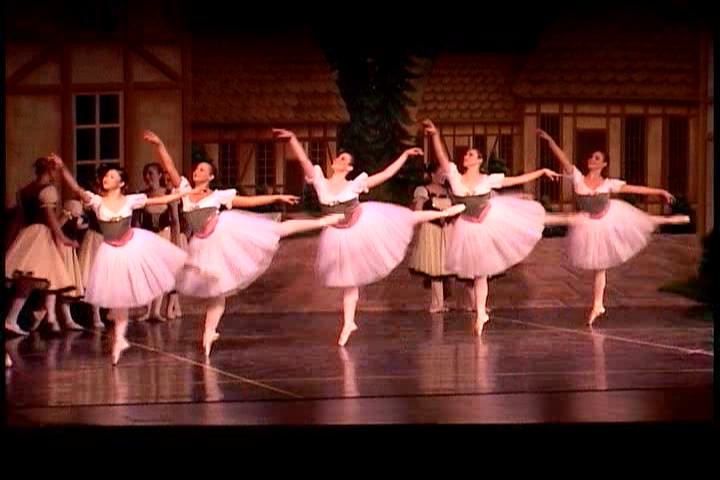On the black performance stage, which beautifully reflects the dancers, a group of five ballet performers captivates the audience with an intricate dance move. Dressed in pink tutus featuring a brown and dark pink design around the midsection, they all gracefully raise their right arms while standing on the tip of their right legs, with their left legs elegantly extended outwards. The stage backdrop depicts quaint, old-fashioned houses and a stone path that stretches across, adding a nostalgic ambiance to the scene. To the left of the stage, a few girls in white skirts and long stockings are seen chatting, providing a charming contrast to the main dance focus.